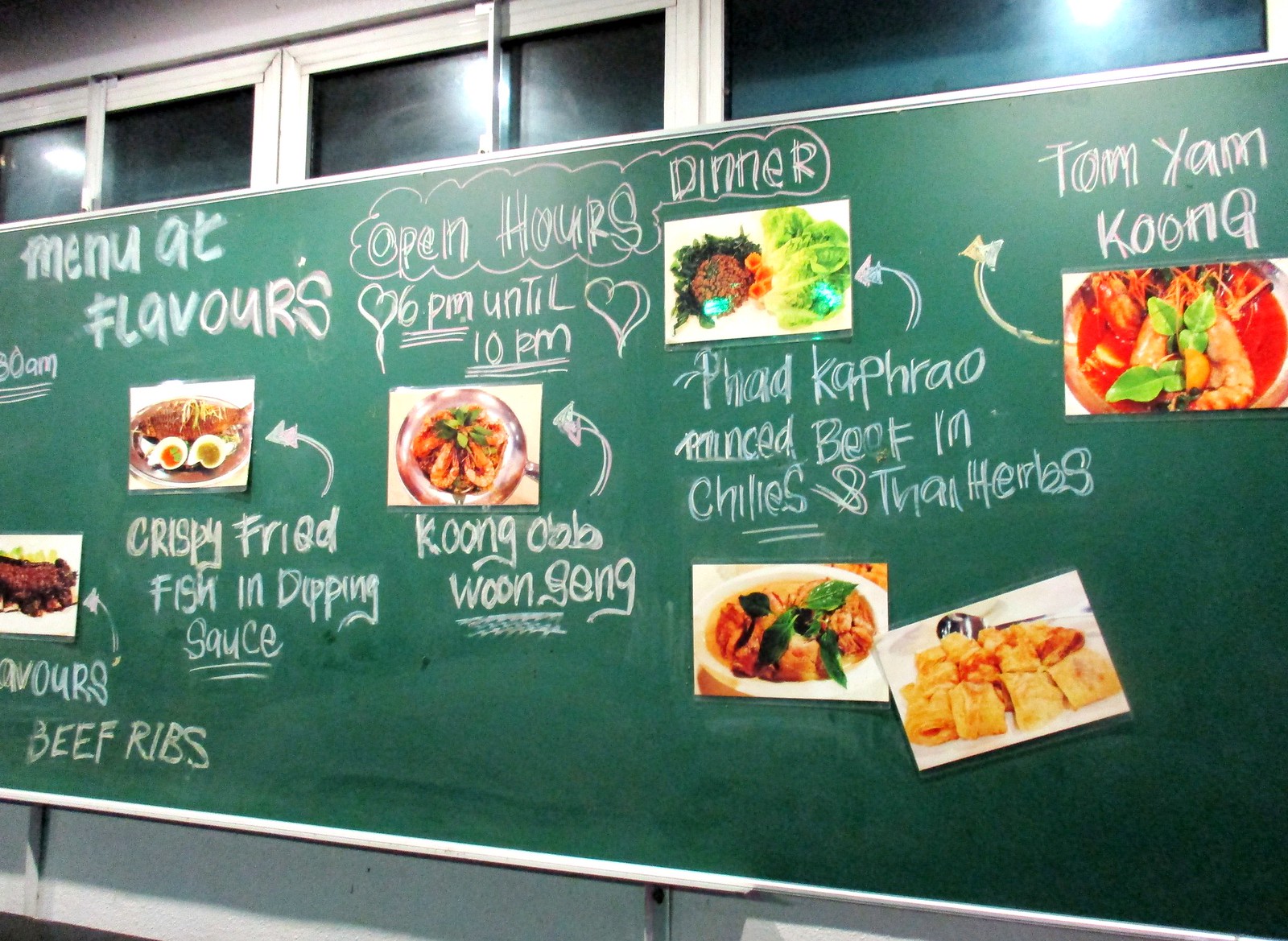The image depicts a large blackboard up against a wall in a restaurant with windows at the top. The main focus is the menu written in chalk, accented with laminated photos of the dishes. At the top left, the board reads “Menu at Flavors” in bubble letters, while the center highlights the open hours, “Dinner, 6 PM until 10 PM”. Surrounding these headings are various dishes with detailed descriptions and arrows pointing to their corresponding images. The dishes include beef ribs, crispy fried fish in dipping sauce, various Thai dishes featuring herbs and chilies, and tom yum kong. Words such as "chilies" and "sauce" are underlined to emphasize key ingredients. The chalkboard serves as a visually engaging display, with labels and photos working together to entice customers.